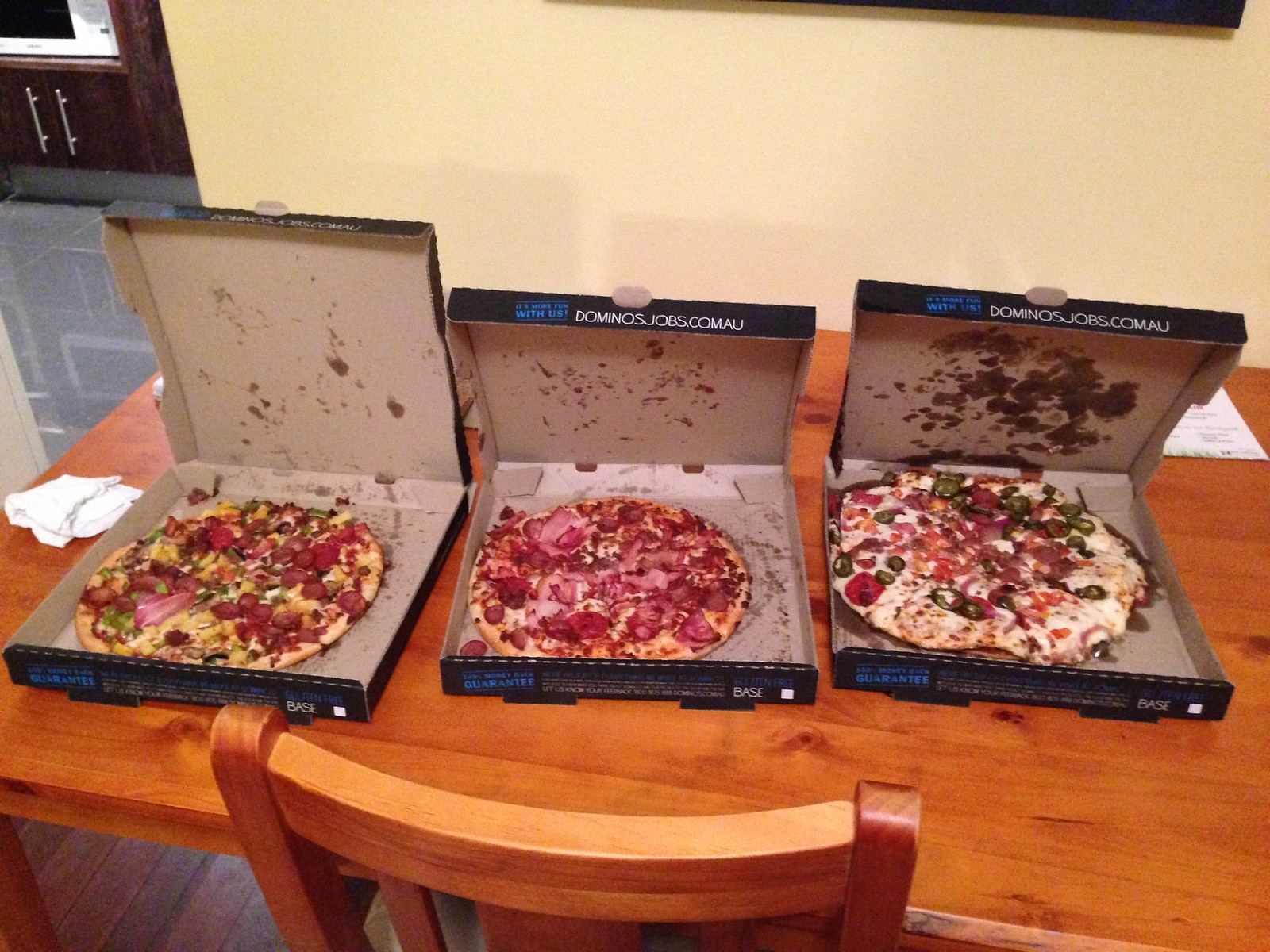This is an image of three open pizza boxes from Domino's, sitting side by side on a light brown wooden desk. The black boxes feature blue and white writing, prominently displaying the URL dominos.jobs.com.au. Each box contains a different type of pizza: a supreme pizza, a ham and cheese pizza, and a pepperoni pizza with jalapenos and black olives. A beige wall serves as the backdrop, with a kitchen cabinet and microwave visible in the shiny reflection of the gray marble floor in the upper left corner. On the desk to the left of the first pizza box, a folded towel is neatly placed. The scene is completed by a wooden chair pushed up to the desk, and a menu can be seen in the background on the right.